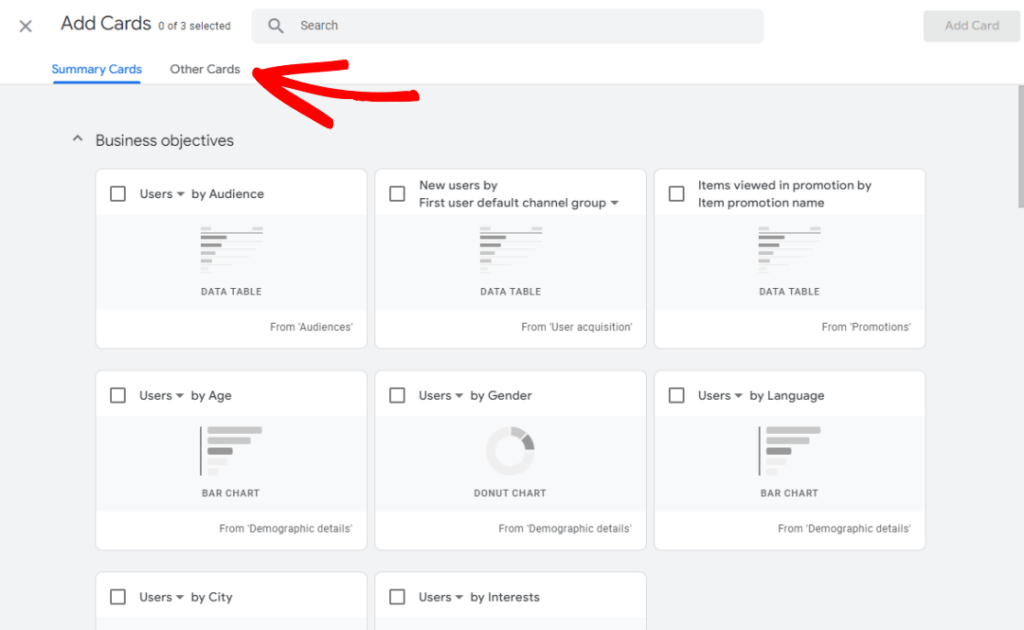A screenshot depicts a user interface designed to add cards, highlighting detailed options for selecting data presentation elements. The area showcases a status of '0 of 3 selected,' with a search bar immediately adjacent and an 'Add Card' button positioned in the upper right corner. Below, there is a segmented section with underlined blue text that reads 'Summary Cards,' which is selected, accompanied by an unselected 'Other Cards' tab. A noticeable hand-drawn red arrow points towards the 'Other Cards' section.

Directly beneath this is a list headed by 'Business Objectives,' followed by an array of panels displayed in a 3x2 grid, although the content extends further down beyond the visible area. Each panel includes a small checkbox to the upper left and corresponding information on the right. None of the checkboxes are marked.

**Detailed Card Descriptions:**
1. **Users by Audience**: Features a simple graphic labeled 'Data Table from Audiences'.
2. **New Users by First User Default Channel Group**: Shows the same graphic, annotated with 'Data Table from User Acquisition'.
3. **Items Viewed in Promotion by Item Promotion Name**: Displays a similar graphic, indicating 'Data Table from Promotions'.
4. **Users by Age**: Depicts a bar chart, described as 'Bar Chart from Demographic Details'.
5. **Users by Gender**: Presents a donut chart, with a partially visible light gray and darker gray striped arc, referred to as 'Donut Chart from Demographic Details'.
6. **Users by Language**: Illustrates a bar chart, also said to be 'Bar Chart from Demographic Details'.

The bottom two panels, labeled 'Users by City' and 'Users by Interests,' have some content obscured and therefore cannot be fully read.

This detailed screenshot captures the intricate layout of the card-adding interface, including visual aids, descriptive labels, and selection features designed to enhance data analysis through various chart representations.